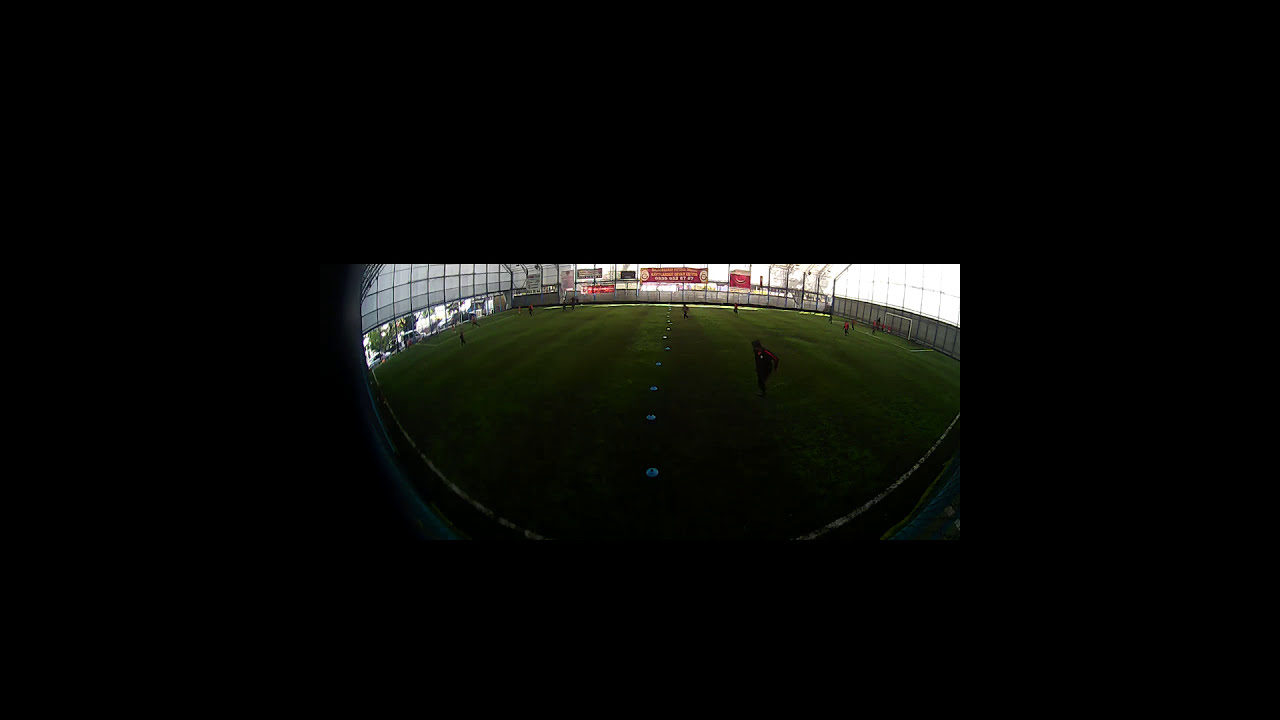This image depicts a soccer stadium captured from an aerial perspective, suggesting a mix of indoor and outdoor elements. The field, characterized by alternating light and dark green stripes, features distinct white markings that highlight the boundaries and centerline of the pitch. The presence of small, blue cones arranged in a straight line suggests a training drill is in progress. Despite the considerable distance, players can be discerned on the field, predominantly donning red and black uniforms, though they appear tiny due to the far-off vantage point. 

Surrounding the stadium is a perimeter fence that appears silver on one side and transitions into a transparent section above it. At the far end, red banners with white and yellow text hang prominently, although the content of the text is not legible. The stadium appears enclosed with large walls composed of grills and blocks, and natural daylight filters through, implying some connection to the outdoor environment. The image itself is outlined in black all around, adding to the sense of depth and framing the vibrant, albeit dimly lit, scene. Trees are visible beyond the fencing, reinforcing the blend of indoor and outdoor aspects of this unique soccer venue.